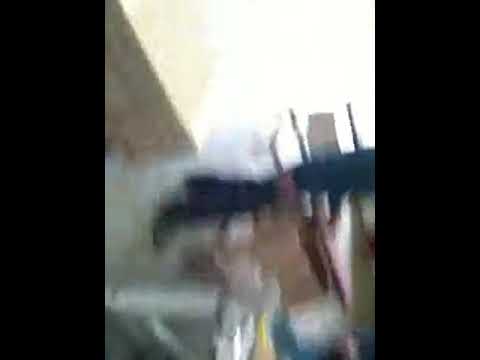The image depicts an extremely blurry scene reminiscent of an abstract painting, making it difficult to discern specific details. The background appears predominantly bright, suggesting the sky, with potential structural elements such as a wall or building on the left side. The middle area is dominated by a dark blue horizontal expanse, possibly representing the horizon, with various shades of gray and dull browns below it. There are several indistinguishable objects protruding from this dark expanse, including something that resembles a brown chimney slightly to the right. On the right and left sides, blocks of black frame the image. The top right corner is notably bright, while the top left has a yellow-tan hue. A diagonal line on the left side descends towards the center, creating a contrast between light beige above and dark brown below. Scattered throughout the image are touches of red, blue, and pinkish elements, adding to the overall abstract and somewhat somber feel of the photograph.